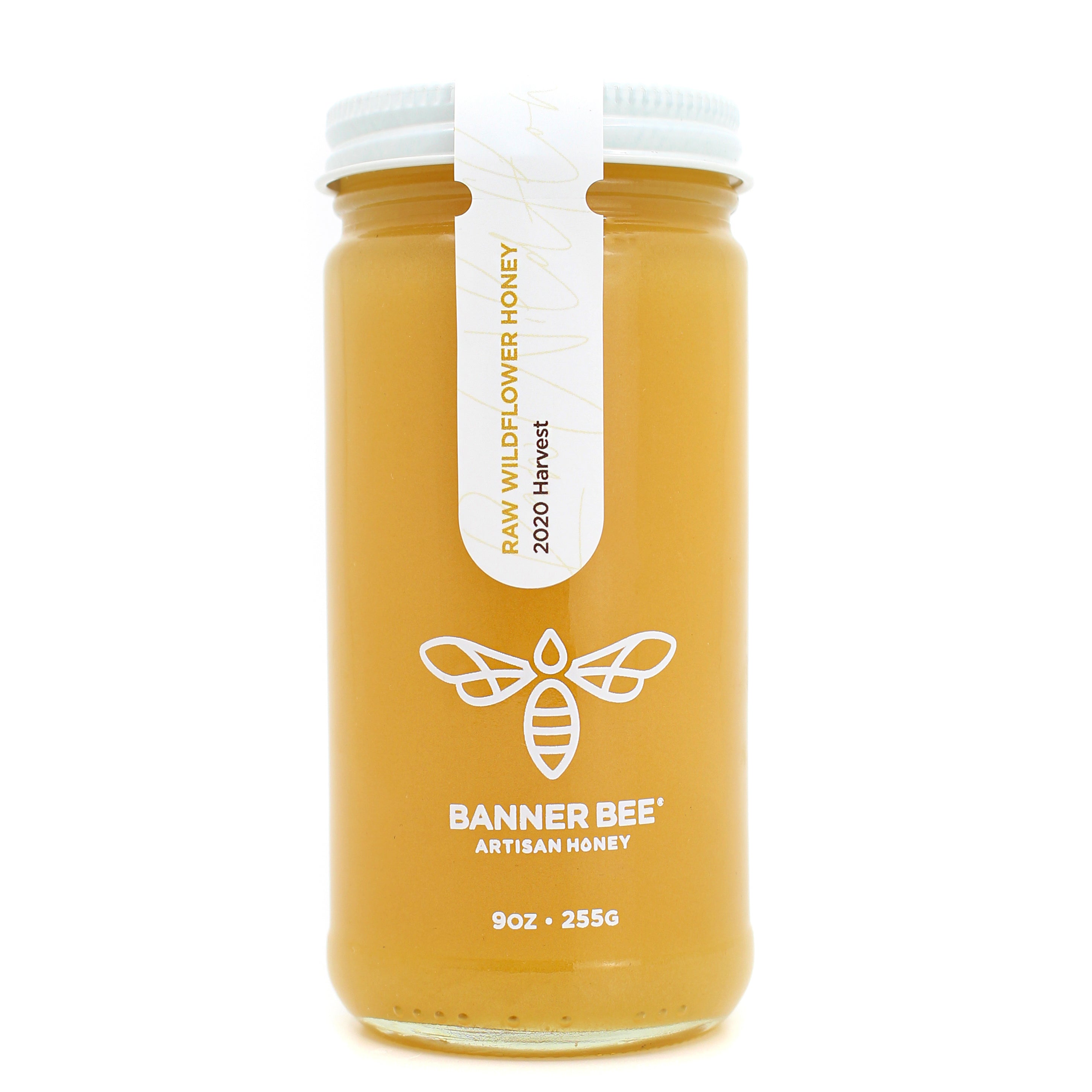This image features a slender, tall jar of Banner Bee Artisan Honey, containing 9 ounces (255 grams) of raw wildflower honey from the 2020 harvest. The jar has a clear, elongated glass body that reveals the golden, slightly murky honey inside. It is sealed with a white metal lid, ensuring that the contents have not been tampered with. A plastic safety label extends from the top of the lid down to the middle of the jar, reading "Raw Wildflower Honey 2020 Harvest" in black font, with "Raw Wildflower Honey" highlighted in a honey-colored ink. The front of the jar showcases a minimalist, white illustration of a bee with distinct outlines for the wings and a teardrop-shaped body, followed by the text "Banner Bee Artisan Honey 9 ounces 255 grams" beneath it. The overall color palette includes various shades of golden yellow, white, brownish-black, light yellow, and gray, enhancing the artisanal and organic aesthetic of the product.